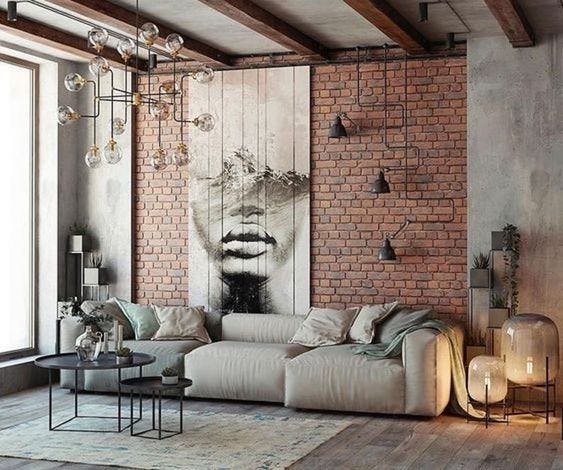This image depicts a stylish, modern living space that combines industrial elements with contemporary art. Located in a big city, likely an apartment, the room exudes a chic, urban vibe. The back wall is constructed with exposed brick, adorned with a large, abstract painting of an African-American woman's face, primarily showcasing her lips and lower half in a blend of intricate patterns. 

A cream-colored sofa with three segments and six pillows in shades of gray, cream, and light seafoam green sits prominently against the brick wall. In front of the sofa, two nesting round tables hold various knickknacks, including vases with plants. 

To the left of the sofa, a floor-to-ceiling window allows soft, gloomy sunlight to filter through, casting a gentle glow around the room. The ceiling, with its dark wooden planks on a beige background, supports a unique, rustic industrial-style chandelier with multiple bulbs. Further emphasizing the industrial motif, the wall-mounted lamp features a metal contraption with three bulbs.

Adjacent to the right end of the sofa, there is a decorative arrangement comprising a large and a small vase, while a plant stand holds four plants, with one cascading gracefully. To the left of the sofa, another plant stand hosts two more plants, enhancing the room's vibrant and organic feel.